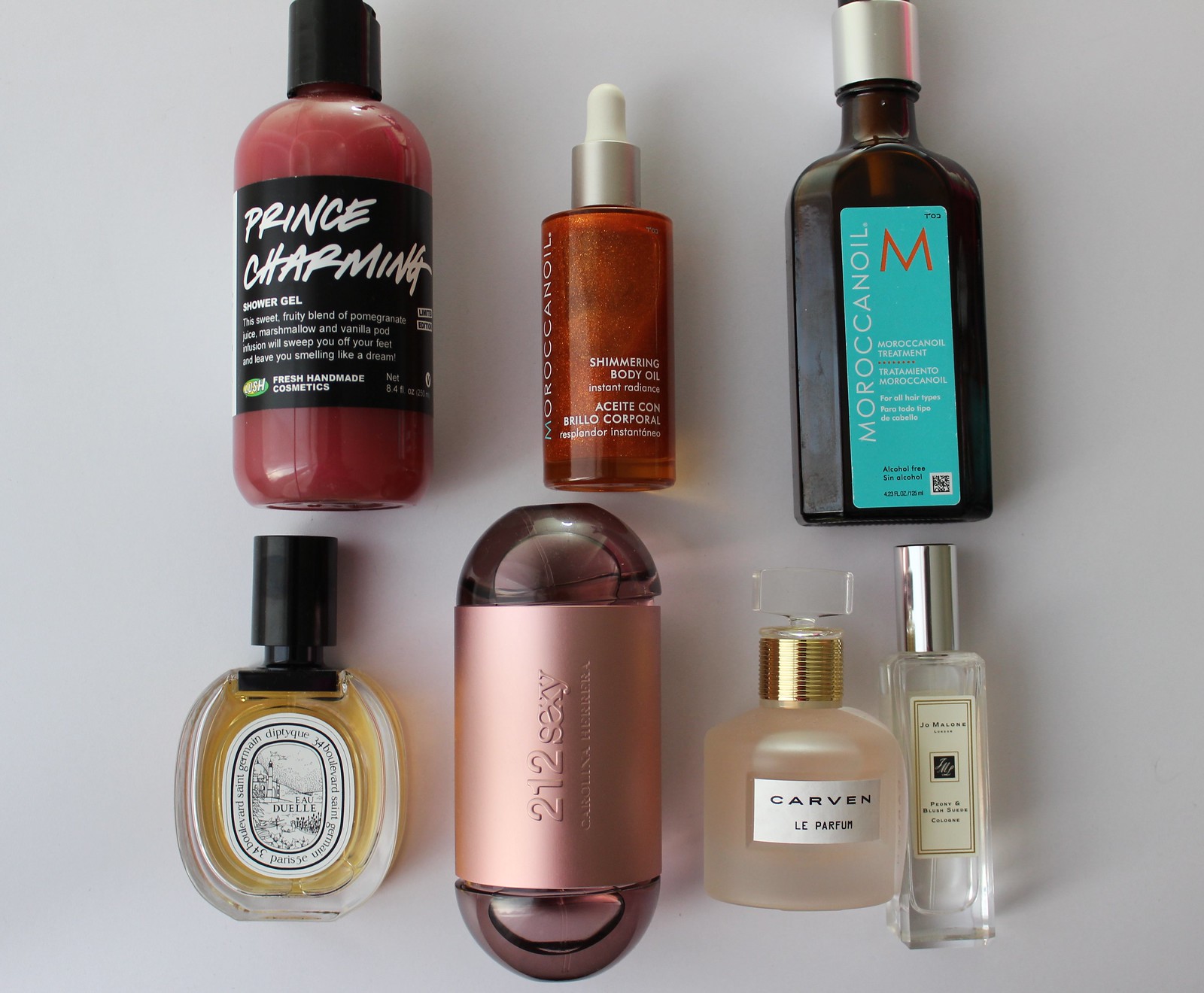The photograph showcases a curated selection of beauty care products against a pristine white background. In the upper left corner, there is a plastic bottle with a black cap and label, containing a reddish liquid called "Prince Charming Shower Gel." Adjacent to it on the right is a brownish bottle with a white dropper top, likely containing body oil. Further to the right, there is a dark brown bottle with a silver cap and a blue label featuring the words "Moroccan Oil" in white, with a prominent orange 'M' at the top.

On the bottom row, starting from the left, there is an oval-shaped glass bottle with a black top, possibly a perfume. To its right is another oval-shaped bottle with a unique, pill-like appearance, featuring a grayish body and a pink label inscribed with "212 Sexy," indicating it is also a perfume. Continuing right, there is a glass bottle with a gold top and a white label that reads "Carbon," suggesting it is another perfume. Finally, on the far right, there is a clear glass bottle with a silver top, which also appears to be a perfume.